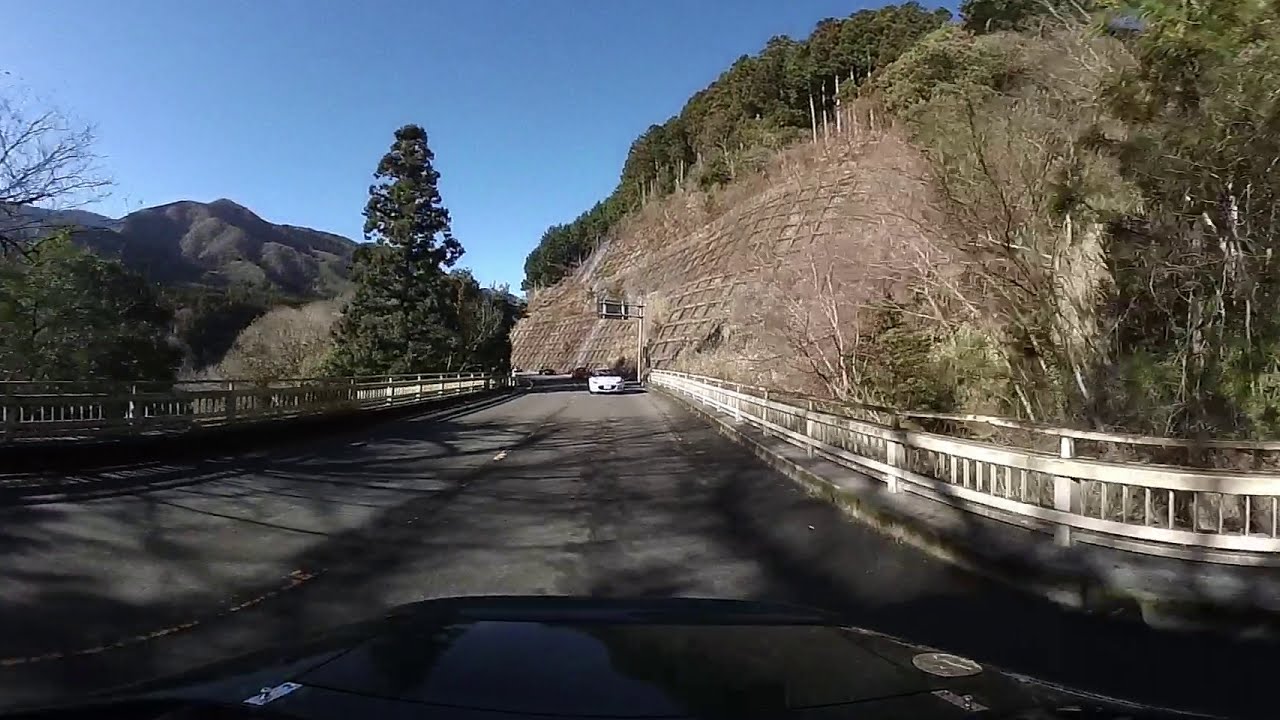The image, taken from the windshield of an unidentified car, captures a serene drive down a two-lane country road that curves gently through picturesque hills. Ahead in the distance, a white car navigates a left turn, while a blue car is also visible on the road. On both sides of the road, white railings reminiscent of picket fences line the route. To the right, a prominent tiered hillside has been reinforced to prevent erosion, displaying a crisscross pattern of ropes or chains. Atop the hillside, dense and immaculate trees stand tall, with pine trees mixed in, hinting at a western locale. On the left side, there's a single tree, adding to the natural beauty. In the background, mountains rise on the right, under a clear blue sky occupying the upper left quadrant, giving the scene a calm, cool atmosphere perfect for a relaxing drive. The overall impression is of a remote, peaceful area with a charming, country vibe.